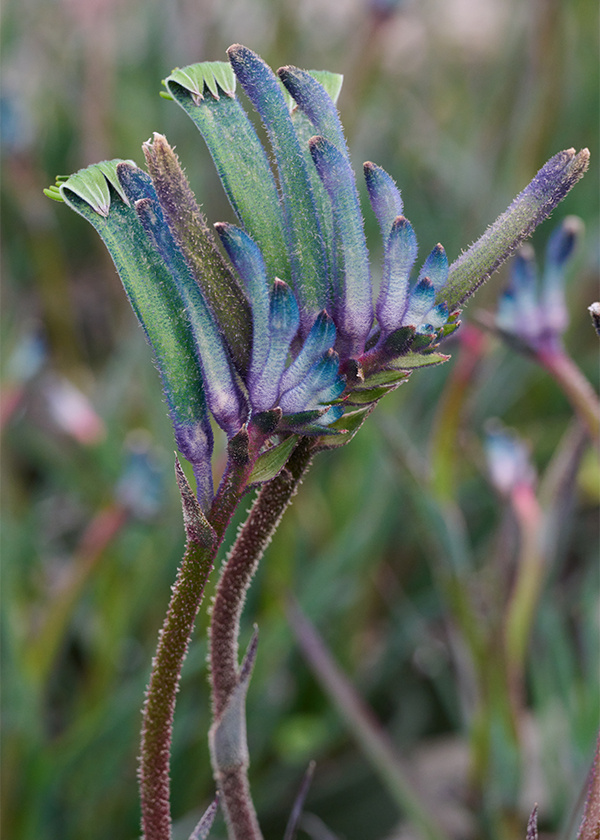This image captures two distinct flowers prominently positioned in the foreground, standing out against a lush, out-of-focus woodland backdrop. The flowers, rising from brown stalks adorned with tiny hair-like features, display an intricate array of green, blue, and purple hues. Each stalk supports leaves that gracefully curl upwards towards the left, middle, and right upper portions of the image. The delicate leaves and flowers encompass a spectrum of colors, adding visual interest. In the background, although blurry, there are noticeable tall grasses and additional similar flowers, particularly on the right side. The setting appears to be deep in the woods, with the periphery characterized by various shades of green and blue, complemented by sporadic touches of purple and tan elements, contributing to the depth and richness of the scene.